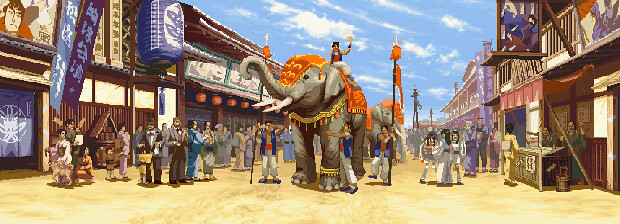In a bustling urban street teeming with onlookers, an elegantly decorated elephant makes its way through the crowd, evoking a scene from a vividly animated or computer-generated illustration. The sky above is a radiant blue with occasional clouds, suggesting a sunny and pleasant day. Japanese signage adorns the buildings, hinting at a possible East Asian setting. Atop the majestic elephant sits a man, confidently waving to the crowd. He is adorned in ceremonial attire, signaling his prominent role in this spectacle. The elephant itself is dressed in ornate orange drapery that covers its head, trunk, and body, enhancing its grandeur. Surrounding the elephant, individuals in blue vests are seen at the front and back, each holding a slender pole topped with an orange flag adorned with points. The scene exudes a celebratory atmosphere, possibly indicating a festive occasion or a wedding procession.